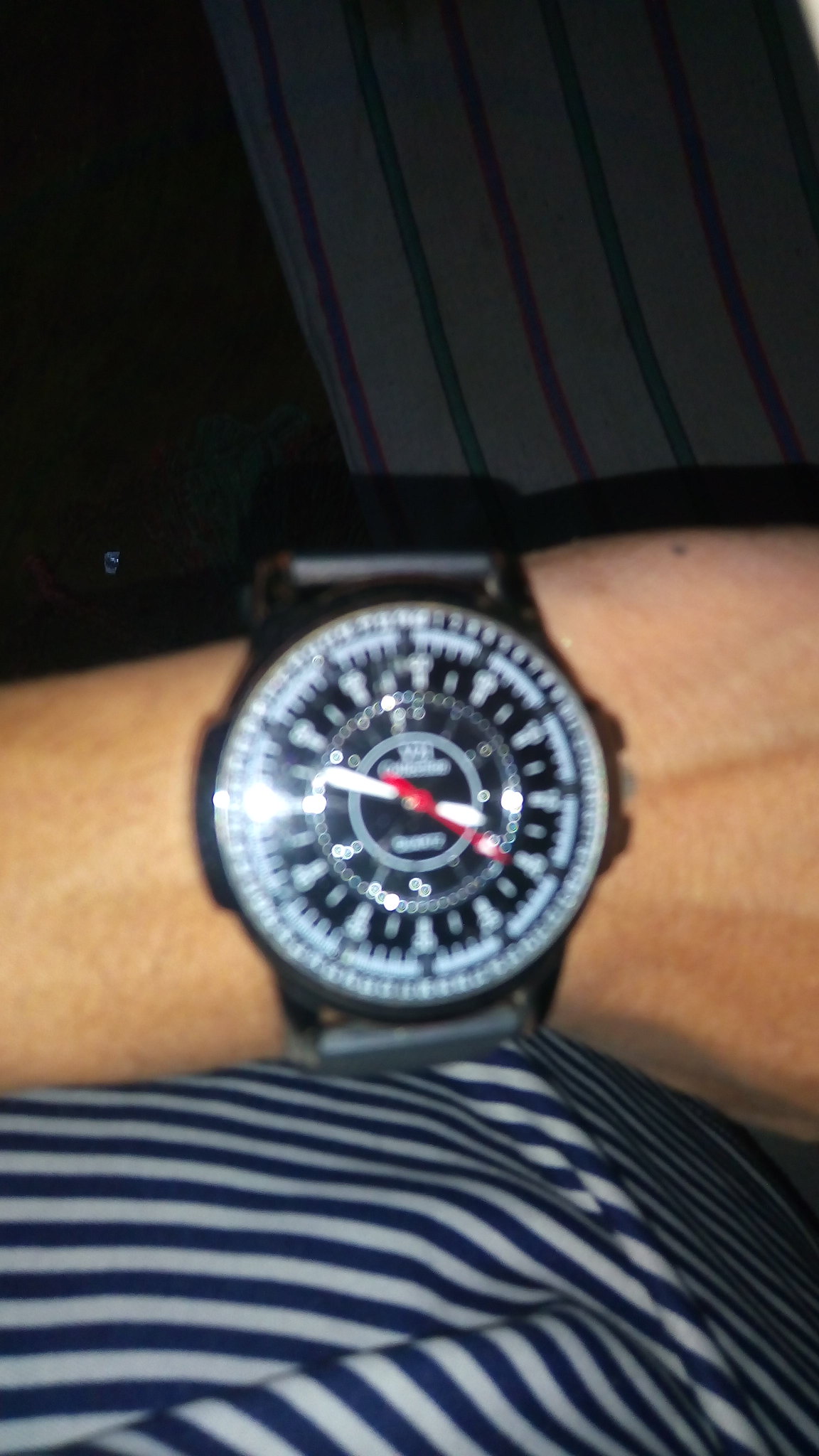In the image, a person is prominently displaying their wristwatch, which is worn on their left wrist. They’re dressed in a blue and white striped shirt with narrow stripes that almost form a V-shape at the center. The room behind them is dark, but the backdrop reveals a lighter, white wall adorned with evenly spaced black lines. 

The wristwatch features a black band and a black face, accompanied by a reflective cover that catches a bit of light. The watch face is detailed with two white hands and a slim red second hand. There are multiple concentric circles on the face, each containing intricate numbers or writing, though they are hard to discern. The numbers around the watch face are in blue and white. Additionally, the person has a distinctive brown mole at the base of their palm.